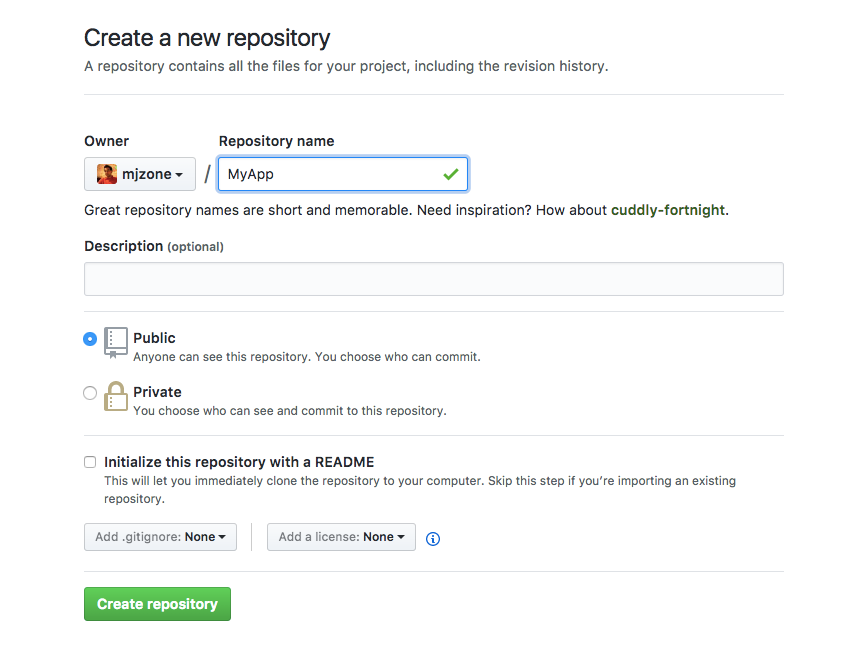The webpage features a stark white background with no margins or boundaries. At the top-left corner, a bold black header reads "Create a New Repository." Directly beneath, in gray text, it explains: "A repository contains all the files for your project, including the revision history." This section is subtly underscored by a faint gray line.

Moving down on the left side, the label "Owner" in black text precedes a dropdown menu with a light blue background. This dropdown displays a specific user, "MJ Zone," accompanied by their profile picture.

To the right, there's a light blue outlined box labeled "Repository Name" in black text. Inside the box, it reads "my_app" with a reassuring check mark to its right. Below this, a note in black text suggests: "Great repository names are short and memorable. Need inspiration? How about Cuddly-Fortnite?"

Further down, the term "Description" is displayed in black text with "(optional)" noted in gray. A long horizontal text box with a light blue background lies empty below this label.

At the bottom, two selection options are presented: "Public" and "Private," both in black text. Under "Public," gray text explains: "Anyone can see this repository. You choose who can commit." Under "Private," it similarly states: "You choose who can see and commit to this repository."